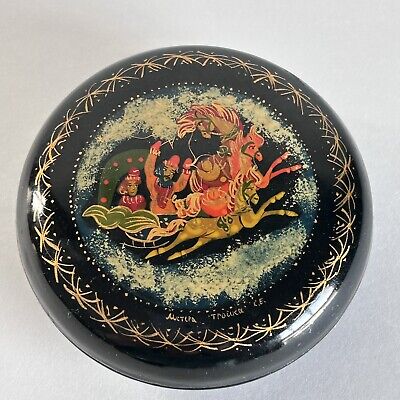The image showcases an intricately designed circular artifact, set against a pale gray background. The object, which appears to be a hand-painted shallow bowl or plate, is primarily black and may be crafted from plastic, glass, ceramic, or painted metal, indicated by the light reflections and material texture.

The outer rim of the artifact features ornate golden X-shaped patterns scattered along the border. Encircling the inner section is a ring of small white dots or squares. This inner portion holds a detailed and vibrant painting, marked by scattered green and yellow swirly clouds. At the core of this scene are three horses of distinct colors: one green, one red, and one tawny brown. Each horse has a flowing mane and is equipped with a saddle.

The central figures in the painting include a bearded man dressed in a pale orange tunic with a red center, wearing a tall orange cap, possibly signifying Middle Eastern or Arabian attire. He is holding the reins of the central, orange horse. Behind him, a woman adorns a headgear and a red costume, seated in what seems to be part of a sled, suggesting they are riding on a horse cart. The overall scene is dynamic, giving the impression that the horses are in motion or flight.

The artifact is signed, with an unreadable signature in gold at the bottom of the painting, lending an air of authenticity and craftsmanship. The mix of stylized patterns and exotic, colorful imagery makes this piece an intriguing decorative item.